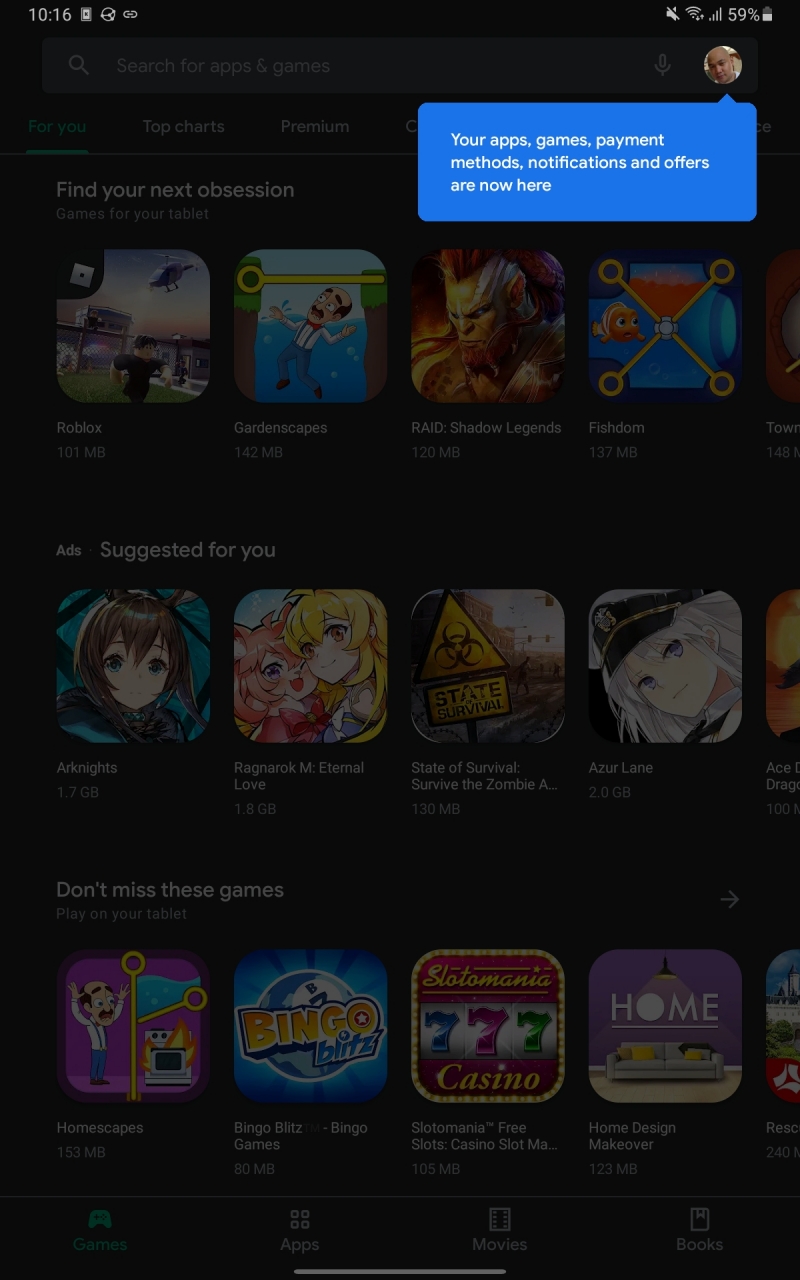A smartphone screen displays a variety of details and notifications. In the top left corner, the time reads 10:16, followed by several status icons that are not clearly identifiable. On the right side of the status bar, you can see the "no sound" icon, cellular signal bars, and a 59% battery charge icon. Additionally, there is a profile photo of a bald individual displaying only their head. A blue notification bubble extends from this profile photo, stating, "Your apps, games, payment methods, notifications, and others are now here."

Below this notification, the screen shows a main display with app icons slightly obscured by a grey overlay. The navigation tabs at the top include "For You," "Top Charts," "Premium," and more, with the "For You" tab highlighted in blue, indicating it is currently selected. A heading under the "For You" section reads, "Find your next obsession," showcasing various game recommendations for the tablet. These game suggestions include:

- Roblox (101 MB)
- Gardenscapes (142 MB)
- RAID: Shadow Legends (120 MB)
- Fishdom (137 MB)

Further down, a section labeled "Ads Suggested for You" lists additional game recommendations with their respective file sizes:
- Arknights (1.7 GB)
- Ragnarok M: Eternal Love (1.8 GB)